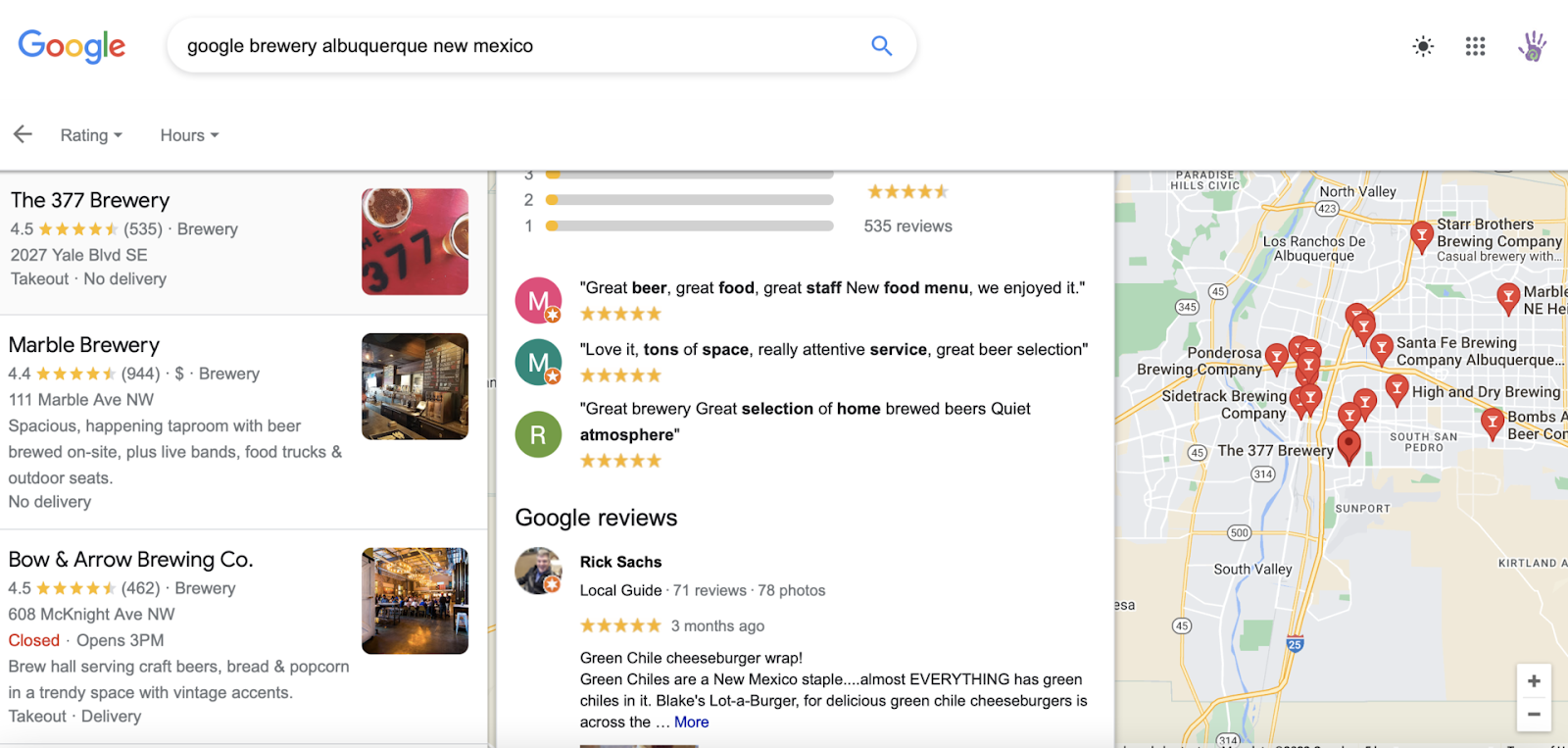A screenshot of Google search results for brewery reviews in Albuquerque, New Mexico. In the upper left corner, the Google search bar contains the query "Google brewery Albuquerque, New Mexico," accompanied by the Google logo. On the lower right, a map showcases multiple brewery locations, marked with red teardrop-shaped pins featuring martini glass icons. Some notable referenced points on the map include 377 Brewery, South Valley, Los Ranchos de Albuquerque, and Star Brothers Brewing Company.

To the left, detailed listings of breweries are visible. The 377 Brewery, located at 2027 Gale Boulevard Southeast, boasts a 4.5-star rating from 535 reviews and is labeled as offering takeout but no delivery. Other entries include Marble Brewery with a 4.4-star rating and Bow and Arrow Brewing Company with a 4.5-star rating. Between the map and brewery listings are user reviews, highlighted by color-coded circles in pink, green, and red with corresponding letters 'M,' 'M,' and 'R.'

One highlighted 5-star review praises the quality of the beer, food, and staff, mentioning a new food menu. Below the main reviews section, "Google reviews" appear in bold black text. A user named Rick Satcha, marked as a local guide with a 5-star review rating, has commented on a green chili cheeseburger wrap, emphasizing that green chili is a staple in New Mexico cuisine. The review hints at more content with an ellipsis and a "more" link in blue.